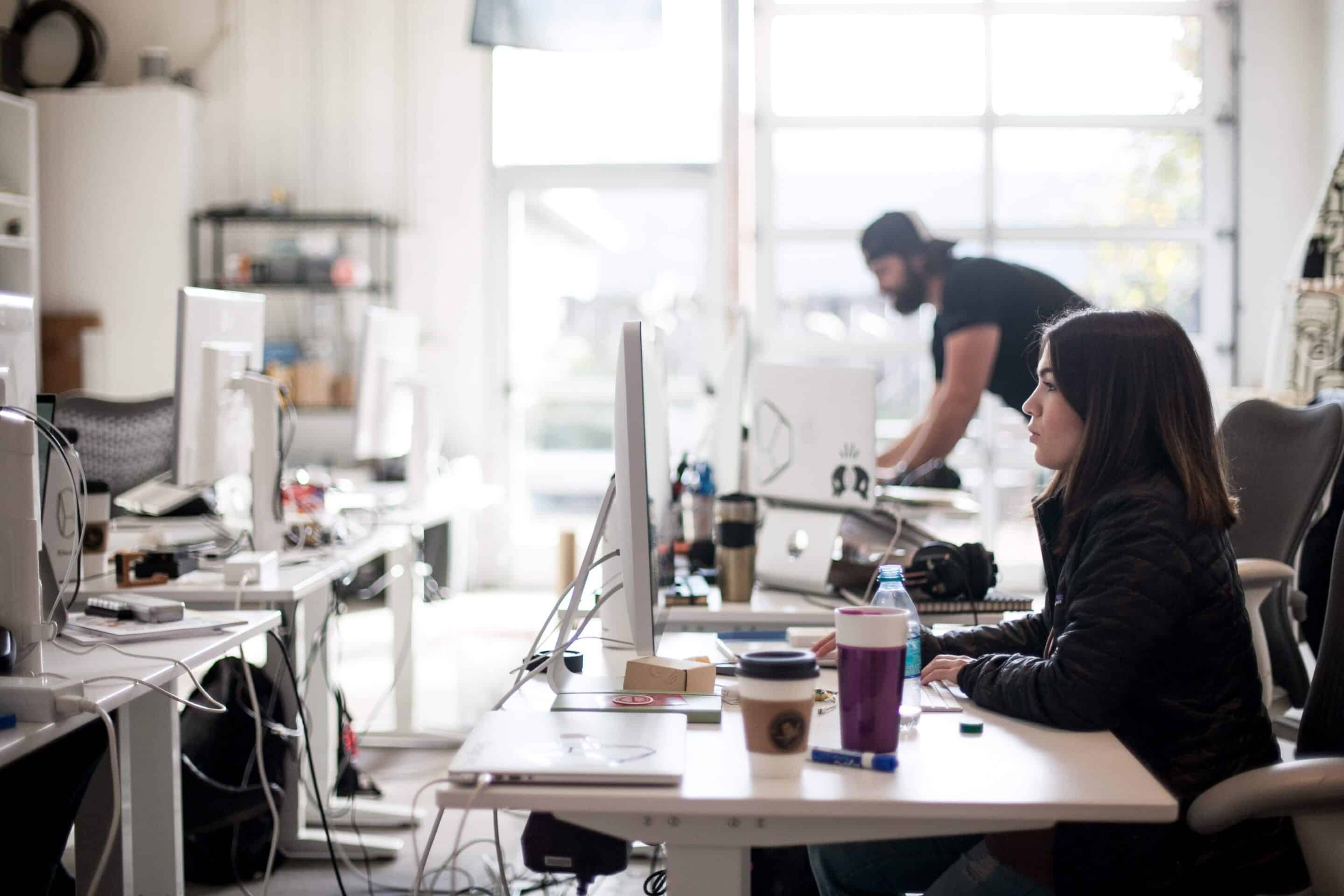In this photograph of a bustling office space, the bright sunlight streams through two large, uncurtained windows, highlighting the white walls and the myriad of desks scattered throughout the room. Various desks are adorned with computers, tangled cords, and personal items, creating a slightly cluttered yet industrious atmosphere. In the foreground to the right, a woman with dark hair, dressed in a black jacket, sits at a desk where multiple items are visible: a closed laptop, a monitor, a travel mug, a coffee cup, a water bottle, and a box. Her hands are poised on the keyboard and mouse as she intently focuses on her screen.

In the background, a bearded man wearing a backwards cap and a black t-shirt leans over a desk, also engrossed in his monitor. He appears to be standing while working, contributing to the dynamic energy of the scene. The room also features light-colored desks, white and possibly black shelves, and some visible backpacks beneath the desks. The image has a slightly blurred background, perhaps intentionally, to draw attention to the diligent workers and their detailed workspace essentials. Overall, it captures a vivid snapshot of a busy and well-lit office environment where both individuals seem deeply engaged in their tasks.